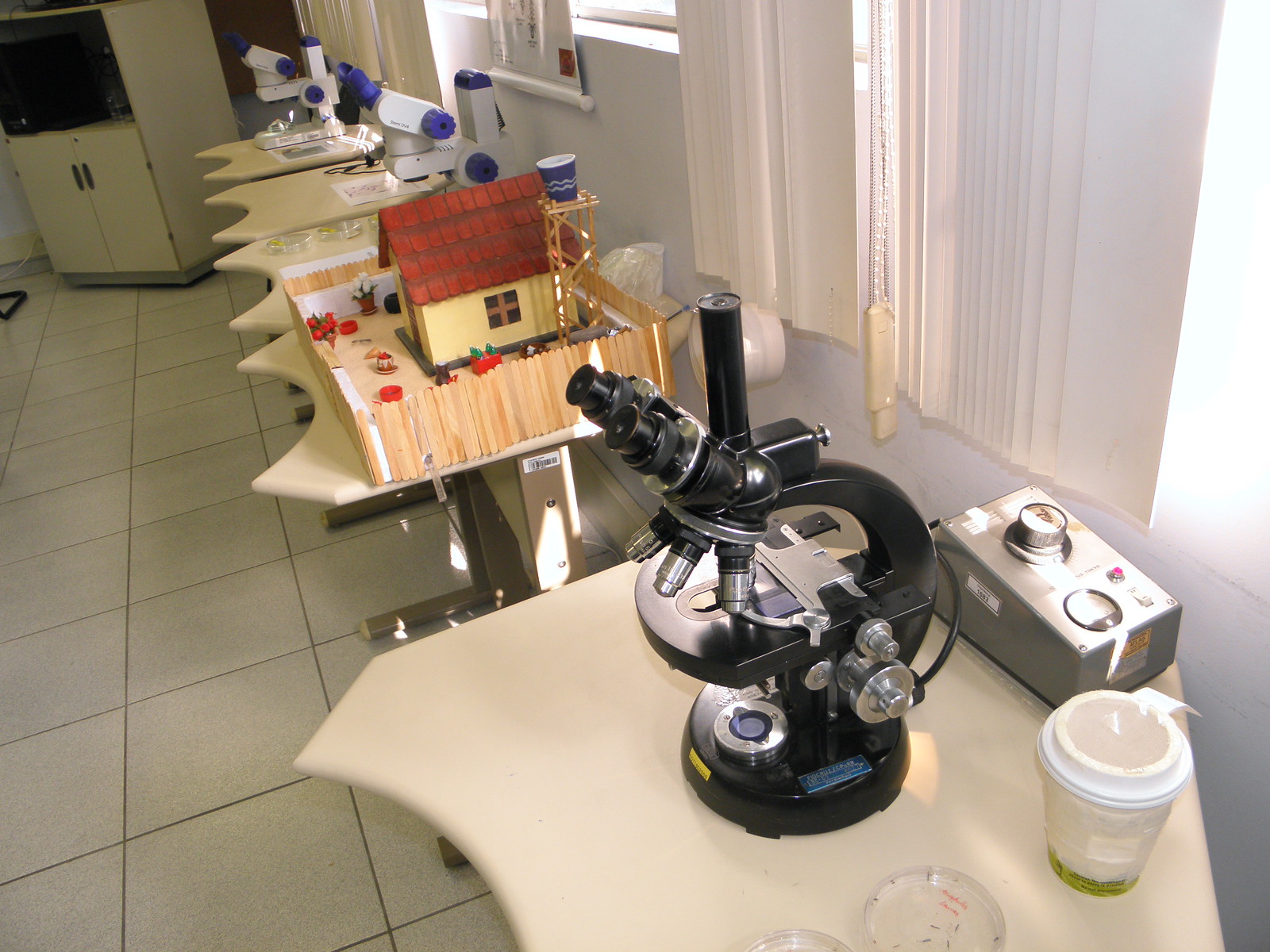The image depicts a brightly lit laboratory or science classroom characterized by its hospital-like aesthetic, with a wall lined with large windows partially covered by drawn open vertical white blinds allowing natural light to fill the room. The flooring consists of white ceramic tiles, enhancing the clean, clinical appearance. Five white trestle-style tables with chrome legs and curved front openings are arranged throughout the room, each tailored for scientific work.

The first table in the foreground holds a microscope, various slides, petri dishes, and a travel coffee cup, suggestive of an ongoing experiment or study. The second table stands out with a detailed diorama featuring a yellow house with a red roof, a popsicle stick fence, a scaffold with a water bucket, and play-doh landscaping, contrasting sharply with the otherwise scientific surroundings. The remaining tables house more microscopes and petri dishes, reinforcing the lab setting.

In the corner of the room sits a tall, rolling cabinet with a video monitor, adding to the functional, academic ambience. This juxtaposition of scientific equipment with a seemingly unrelated diorama hints at a multifaceted use of the space, potentially blending academic lab work with student projects or creative displays.